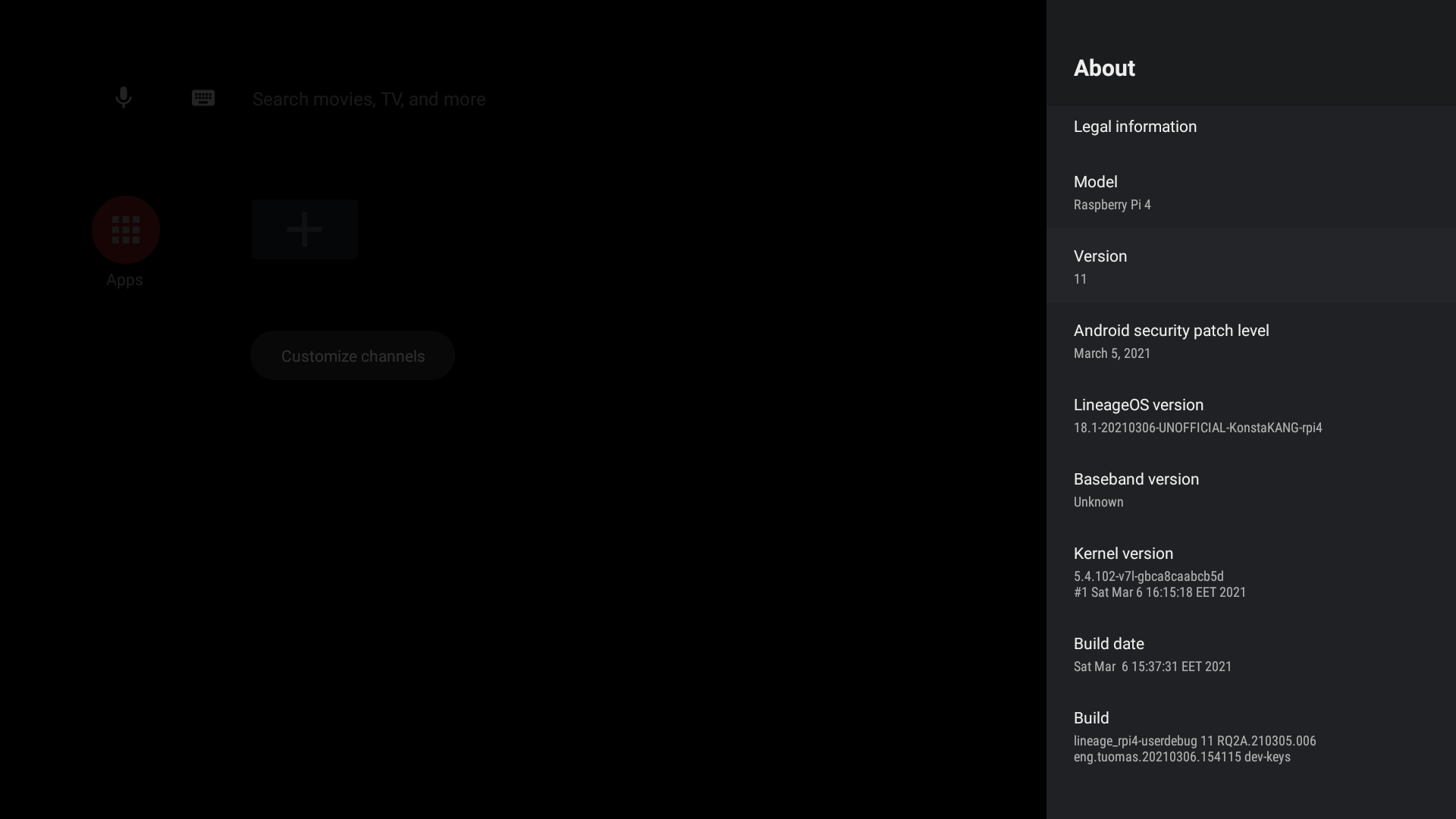The image showcases a web page displayed against a solid black background, with the majority of the page consisting of empty black space. On the right side, there is a vertical block of text providing detailed information about a device. At the top, in bold white text, it reads "About." Below it, in smaller white text, are the sections "Legal Information" and "Model: Raspberry Pi 4." Next, in bold, is "Version: 11." Further down, it mentions "Android security patch level: March 5th, 2021." This is followed by "LineageOS version: 18.1-20210306-unofficial-CostaKang-RPI4." Beneath these entries, additional details include "Baseband version," "Kernel version," "Build date," and "Build number."